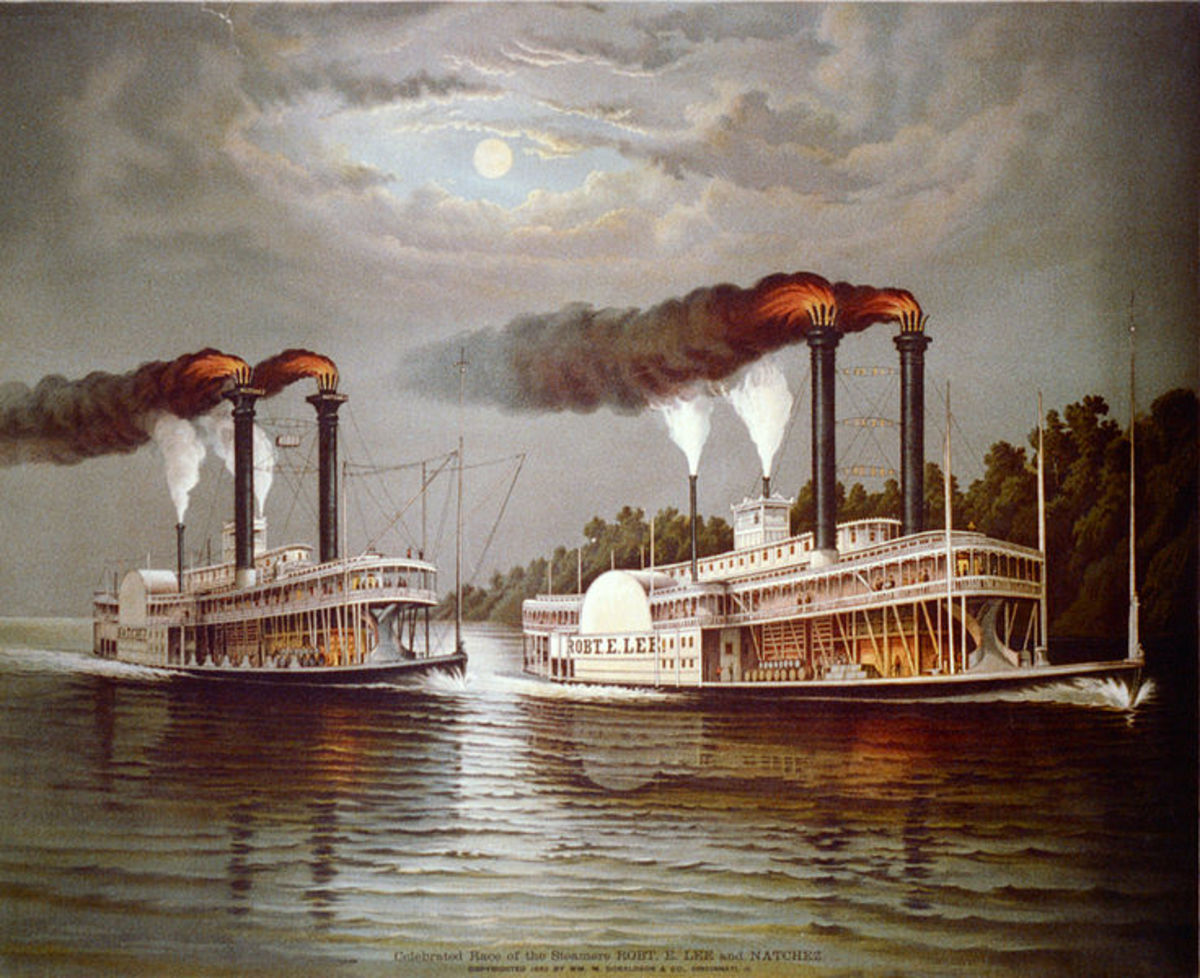The painting titled "Celebrated Race of the Steamers Robert E. Lee and Natchez" vividly depicts two iconic 19th-century American paddlewheel steamers engaged in an intense race on a wide river, possibly the Mississippi. Both majestic vessels, white with gilded accents, have towering twin black smokestacks emitting vivid flames and thick charcoal smoke, with additional smaller funnels expelling white steam. The steamboats, the Robert E. Lee and the Natchez, are shown charging ahead side-by-side, creating waves on the reflective, brownish water. The decks of the steamers are bustling with details, showing passengers, barrels, and dry goods, contrasting with the natural tranquility of the backdrop. The right bank of the river is lined with a tapering row of green-leafed trees, providing a boundary to the scene. Above, the dramatic sky is filled with swirling grey clouds, partially clearing to reveal a small, bright moon, casting a bluish hue across the evening scene, enhancing the sense of an ongoing race under the twilight.